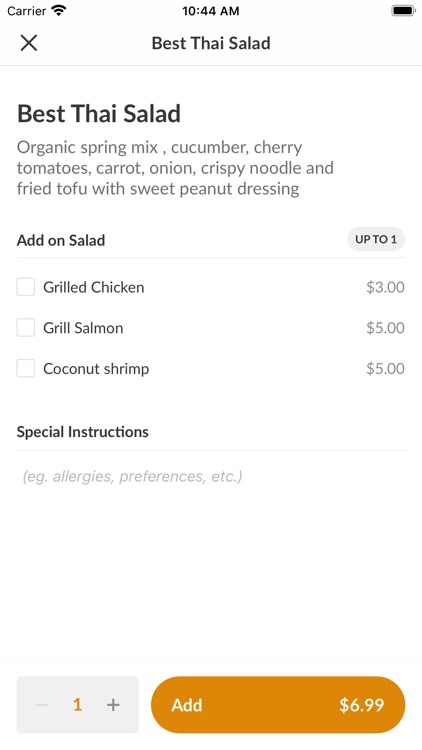A smartphone screen displaying a food ordering app is featured in the image. The status bar at the top shows the carrier, full Wi-Fi signal, the time as 10:44 AM, and a fully charged battery. Below the status bar, an 'X' is seen in the upper left corner, suggesting an option to close the menu.

Centered on the screen is the title "Best Thai Salad," which is described as a mix of organic spring greens, cucumber, cherry tomatoes, carrot, onion, crispy noodles, and fried tofu, all drizzled with a sea peanut dressing. 

Additional options for protein add-ons are available: grilled chicken for three dollars, grilled salmon for five dollars, or coconut shrimp for five dollars. 

Near the bottom of the screen, there is a section for "Special Instructions" where additional notes for the order can be typed. 

At the very bottom, a gray box with an orange number indicates the quantity of one, and an orange 'Add’ button with a price of $6.99 is prominently displayed.

The overall aesthetic features a white background with black text, providing a clean and user-friendly interface.